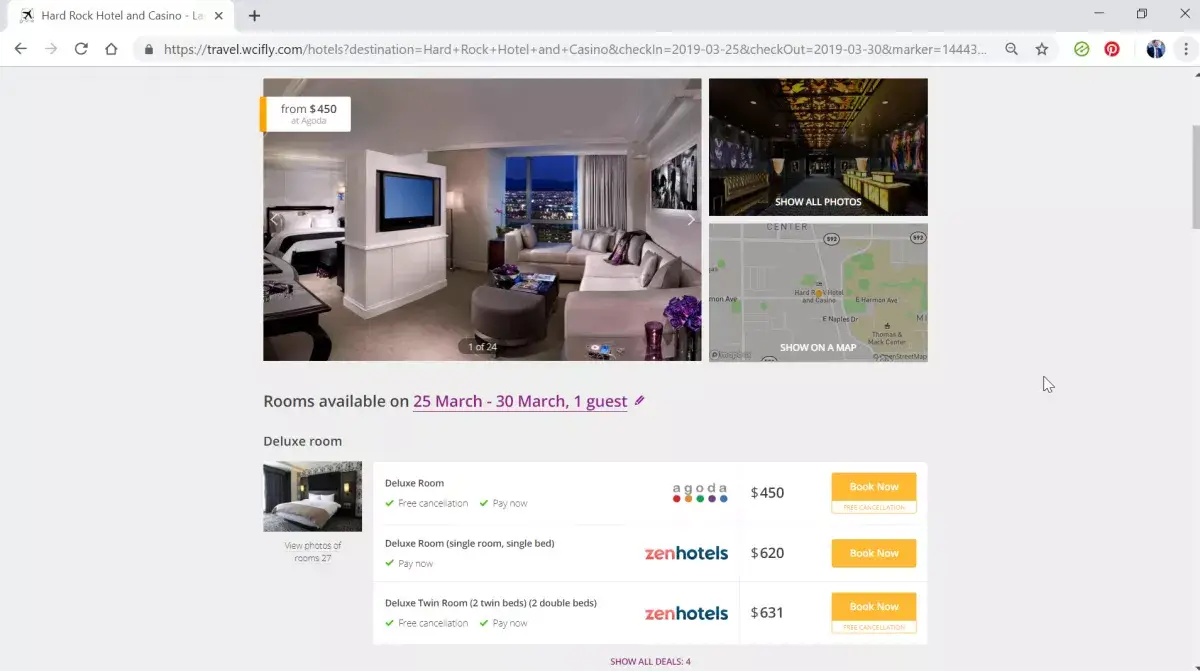This screenshot captures a travel website focused on the Hard Rock Hotel and Casino. At the top left corner, a prominent tab labeled "Hard Rock Hotel and Casino" is displayed. Adjacent to it on the left, there's a gray banner featuring navigation icons for seamless browsing within the site. The layout suggests a user-friendly design typical of travel websites. 

The main section showcases vibrant photographs of the lavish rooms available for booking and enticing images of the casino, offering a glimpse into the luxurious accommodations and thrilling gaming experiences one can expect. A detailed map is also featured, assisting visitors in locating the hotel and casino. Below the visual content, the website provides comprehensive information about room availability and purchasing options, ensuring potential guests have all the details needed for an informed booking decision.